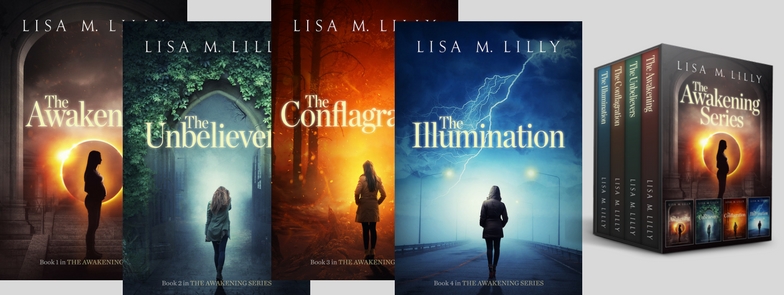The image features a wide, rectangular photograph with a solid medium gray background, no border, and colorful elements. On the left, four book covers by author Lisa M. Lilly are slightly stacked atop one another, showcasing their vibrant designs. The first book, "The Awakening," displays a silhouette of a woman standing before a yellow sun against a dark, brown-black backdrop. The second book, "The Unbeliever," features a woman walking towards an ivy-covered arch, possibly a church entrance. The third book, "The Conflagration," shows a woman standing in front of a forest fire, engulfed in intense orange and red hues. The fourth book, "The Illumination," captures a woman walking down a highway lined with lights under a stormy sky, with lightning piercing through shades of blue and white.

On the right side of the image, a boxed set of the four books is presented, arranged diagonally to display their spines clearly. The cover of "The Awakening" is prominently shown at the front of this stack. Above the set, "The Awakening Series" is written in large, gold-colored letters, along with the author's name, Lisa M. Lilly, placed above an image of a silhouetted woman standing in front of a sun, likely correlating with the cover of the first book. This composition likely serves as an advertisement for the complete series, emphasizing the continuity and thematic elements across the covers.